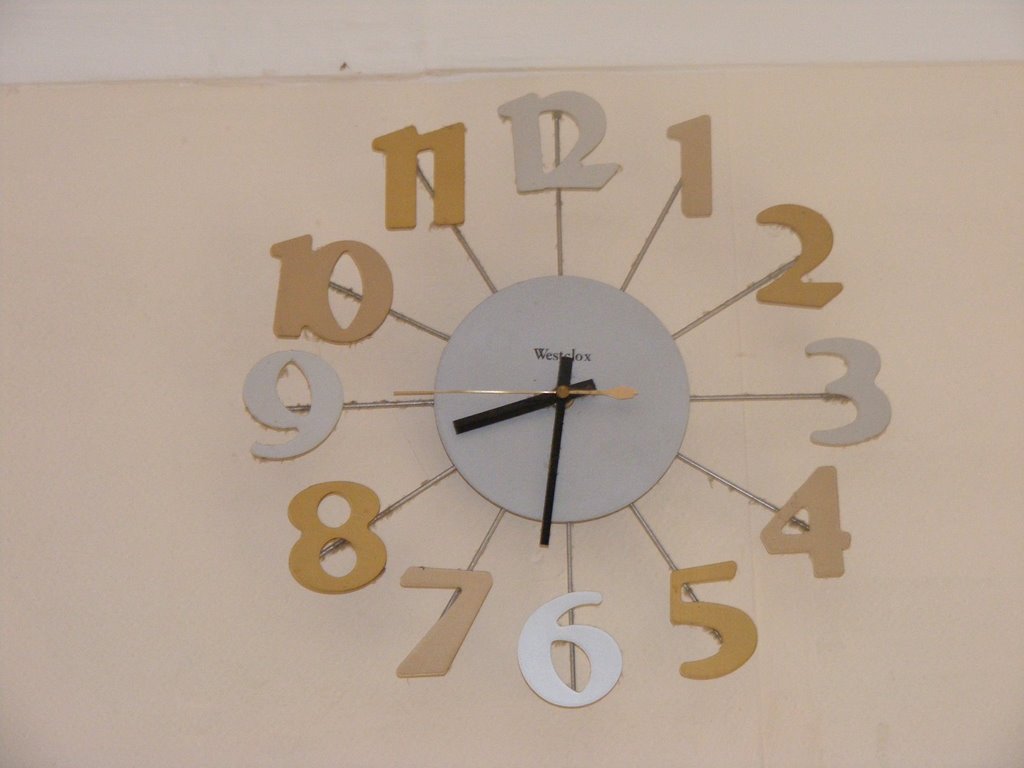This image showcases a wall clock hanging on a peach-colored wall. At the top of the image, the wall transitions to a lighter beige or cream color, likely indicating the ceiling, though the exact boundary is unclear due to image cropping. A dark crack appears to run through the wall at the junction where the colors change, but the precise angle of the cream section remains indeterminate.

The clock itself is small and round, featuring what appears to be a metal plate. Radiating from the center are thin rods that extend to where silver and gold numbers are attached, marking the hours. The clock hands consist of black hour and minute hands, and a gold second hand. The clock's face bears the brand name "Westclox" in black letters, indicating the manufacturer.